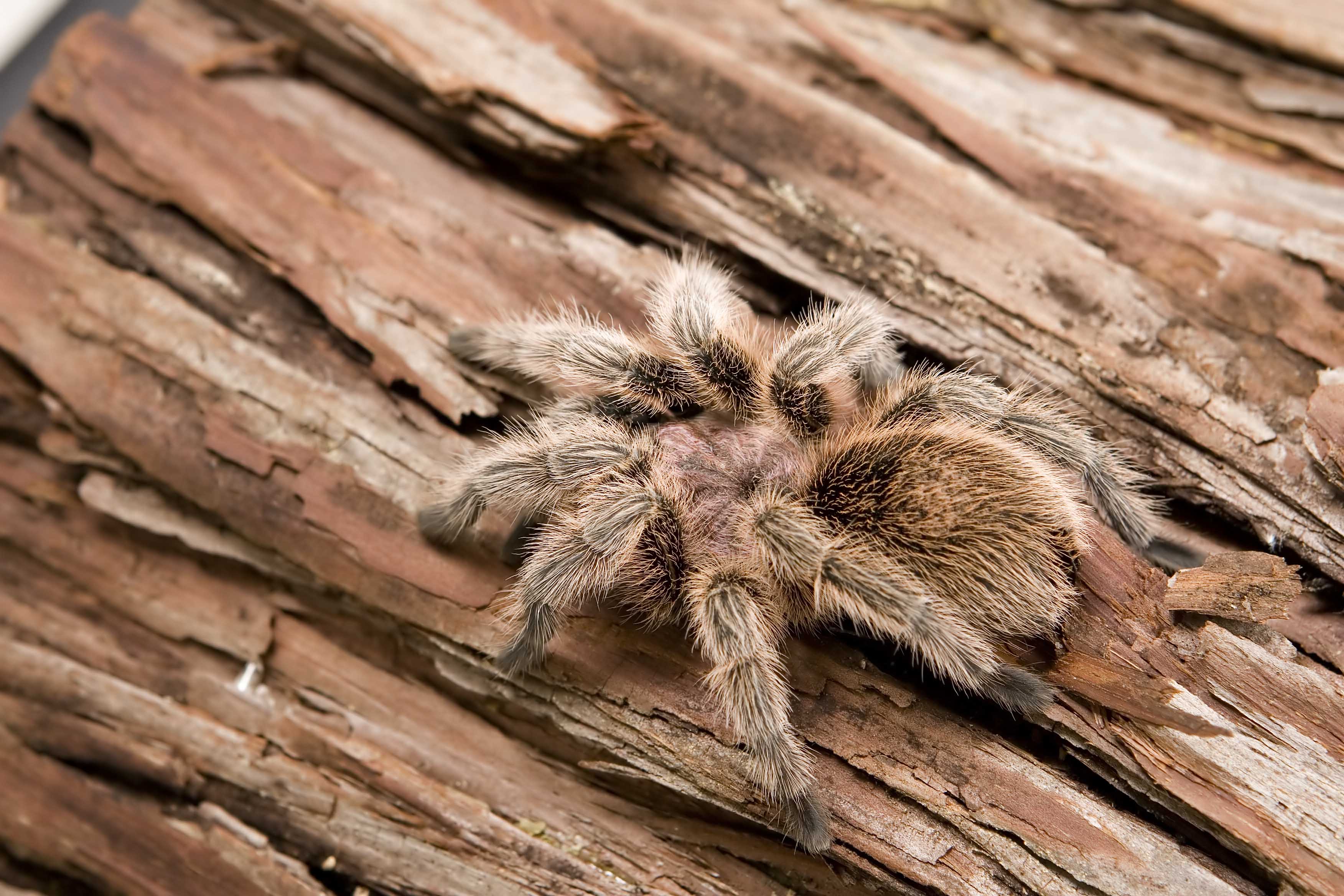The close-up image captures a large, furry spider on a textured wooden surface. The wood's grain, characterized by a series of uneven, parallel brown lines, runs diagonally from the upper left to the lower right of the frame, resembling a tree trunk. The spider, centrally positioned and unmistakable, boasts a detailed appearance: it is predominantly brown with light brown, hairy legs that have dark tips. Its body features darker hairs, particularly on the oval-shaped posterior. Notably, there's a small patch of red in the center of its body. The spider appears to be moving from the lower right towards the middle left, enhancing the dynamic feel of the composition.